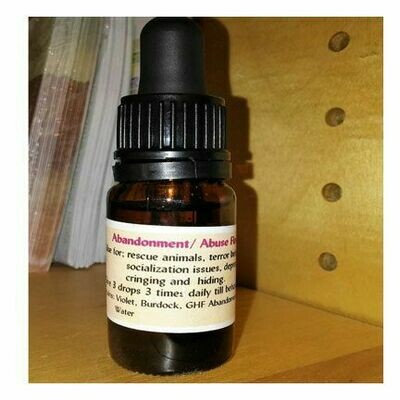The image displays a small, dark brown glass dropper bottle, commonly used for administering medicine. The bottle features a black lid with a rubber squeeze top. An off-white label wraps around the bottle, making some text difficult to read. The label has purple text at the top that reads "abandonment/abuse" and below that, in black text, it includes phrases like "for rescue animals," "terror," "socialization issues," "cringing and hiding," and instructions for dosage: "three drops three times daily." The bottle is positioned on a wooden bookshelf, which has visible notch holes on the right side and papers placed behind it.